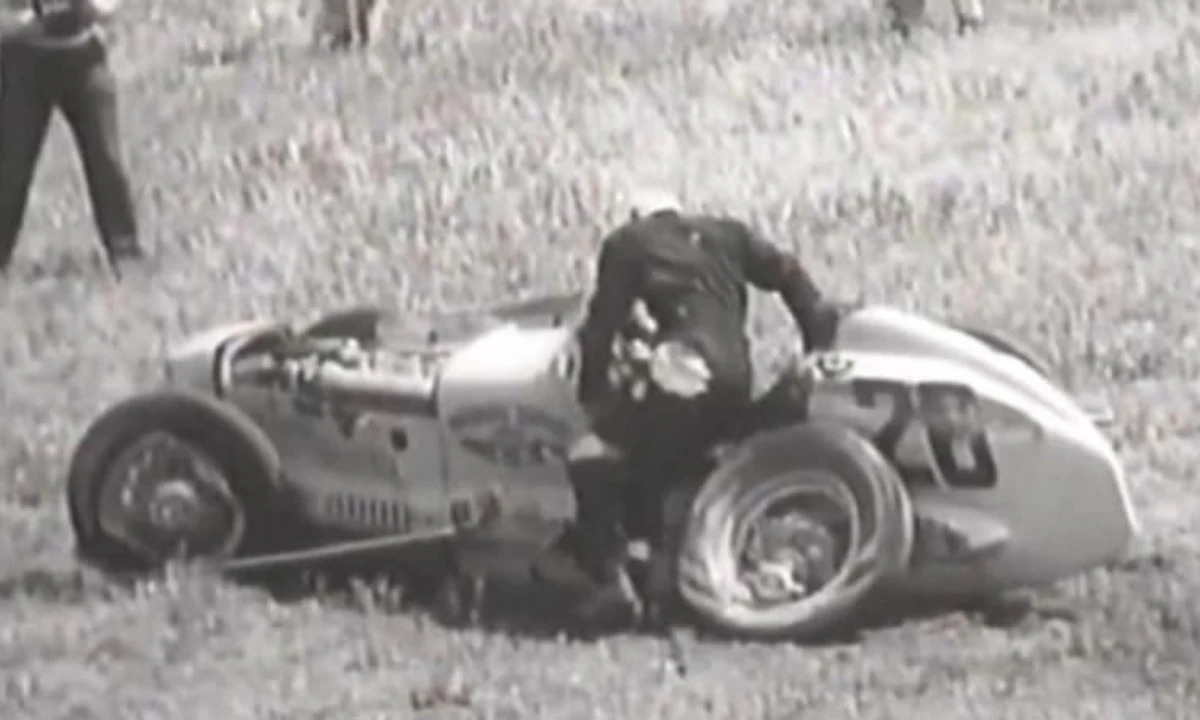In this grainy black and white photograph, seemingly taken outdoors during a race in the 1950s, an old roadster race car with the number 26 prominently displayed on its side lies crashed in a grassy field. The car, possibly a one-seater or two-seater, has one of its wheels completely deformed and ripped off, propped against the car in a testament to the severity of the wreck. The roadster, with exposed motors and likely adorned with advertising, showcases the typical design of racing hot rods from that era. A man, wearing a helmet and a racing jumpsuit with noticeable burn damage on its back, is seen climbing out of the driver’s seat, suggesting he has just survived the wreck. In the background, to the upper left, stand several people, possibly from the press, their legs and cameras partially visible, capturing the scene of the crash. This evocative image captures not just a moment of misfortune but a glimpse into the storied past of vintage automobile racing.